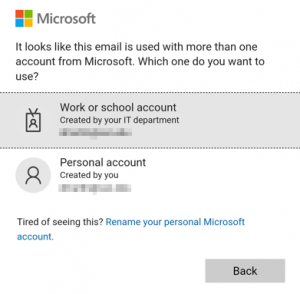The image depicts a Microsoft Outlook prompt presented on a white background. In the top left corner, the Microsoft name and Windows logo are prominently featured. Below this, a message reads: "This email address is associated with multiple Microsoft accounts. Which one would you like to use?"

Two selectable options are presented:

1. The first option, which is highlighted in a darker gray to indicate it has been selected, reads: "Work or school account created by your IT department," adorned with a small briefcase icon to its left.
2. The second option, displayed in regular gray, reads: "Personal account created by you," and is accompanied by an outline of a person icon.

Below these options, a line of text states, "Tired of seeing this?" followed by a blue hyperlink that says, "Rename your personal Microsoft account." At the bottom right corner of the image, there is a radio button labeled "Back."